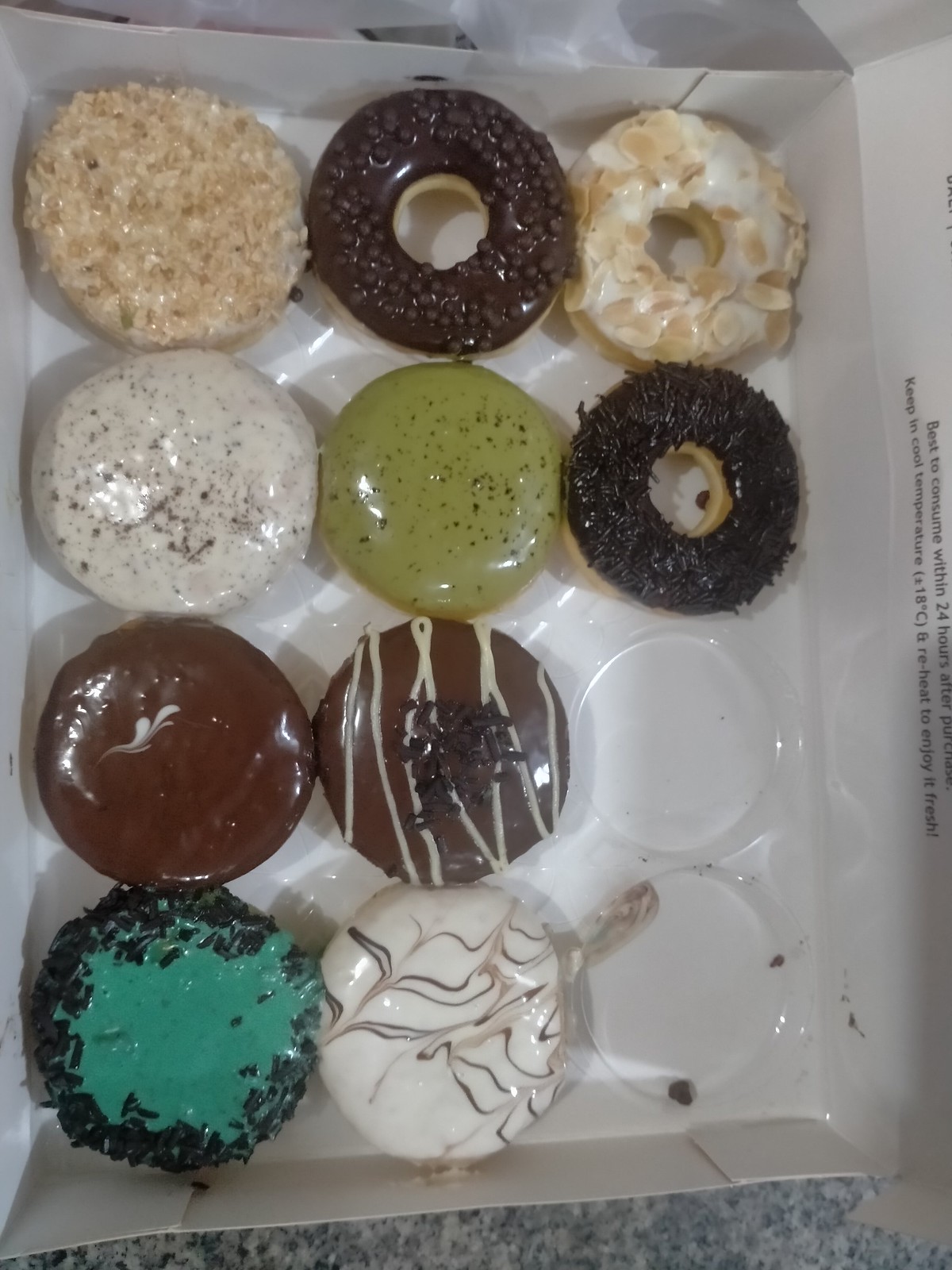This image captures a close-up view from above into a white cardboard box, which originally held a dozen donuts but now contains only ten, with two missing in the bottom right corner. The box's top flap bears an advisory in black text, reading "Best to consume within 24 hours after purchase. Keep in a cool temperature (+/- 18 degrees Celsius) and reheat to enjoy fresh!" The remaining donuts, each nestled in a plastic liner with small holes, display a variety of vibrant colors and toppings.

Starting from the top left and moving right, the first donut features white icing with streaks of chocolate drizzle. Beside it is a chocolate brown donut adorned with dark chocolate shavings and a zigzag of white icing. Next is a milk chocolate donut, accentuated with what appears to be white icing formed into small petal shapes. The donut following that one seems to be coated with chocolate and coconut shavings.

Continuing to the second row, the first donut is olive green with black specks. Next is a white iced donut sprinkled with black flecks. Moving right, the following donut has white icing topped with either coconut or similar shavings. The last donut in this row is chocolate covered with small, chocolate-colored beads on top.

In the third row, the first donut has a white opaque glaze with beige shavings, while the next donut is absent, revealing the empty space in the bottom right corner where two donuts are missing.

Overall, these remaining donuts, with their diverse and elaborate designs, make for an enticing and colorful display, almost too appealing to resist.